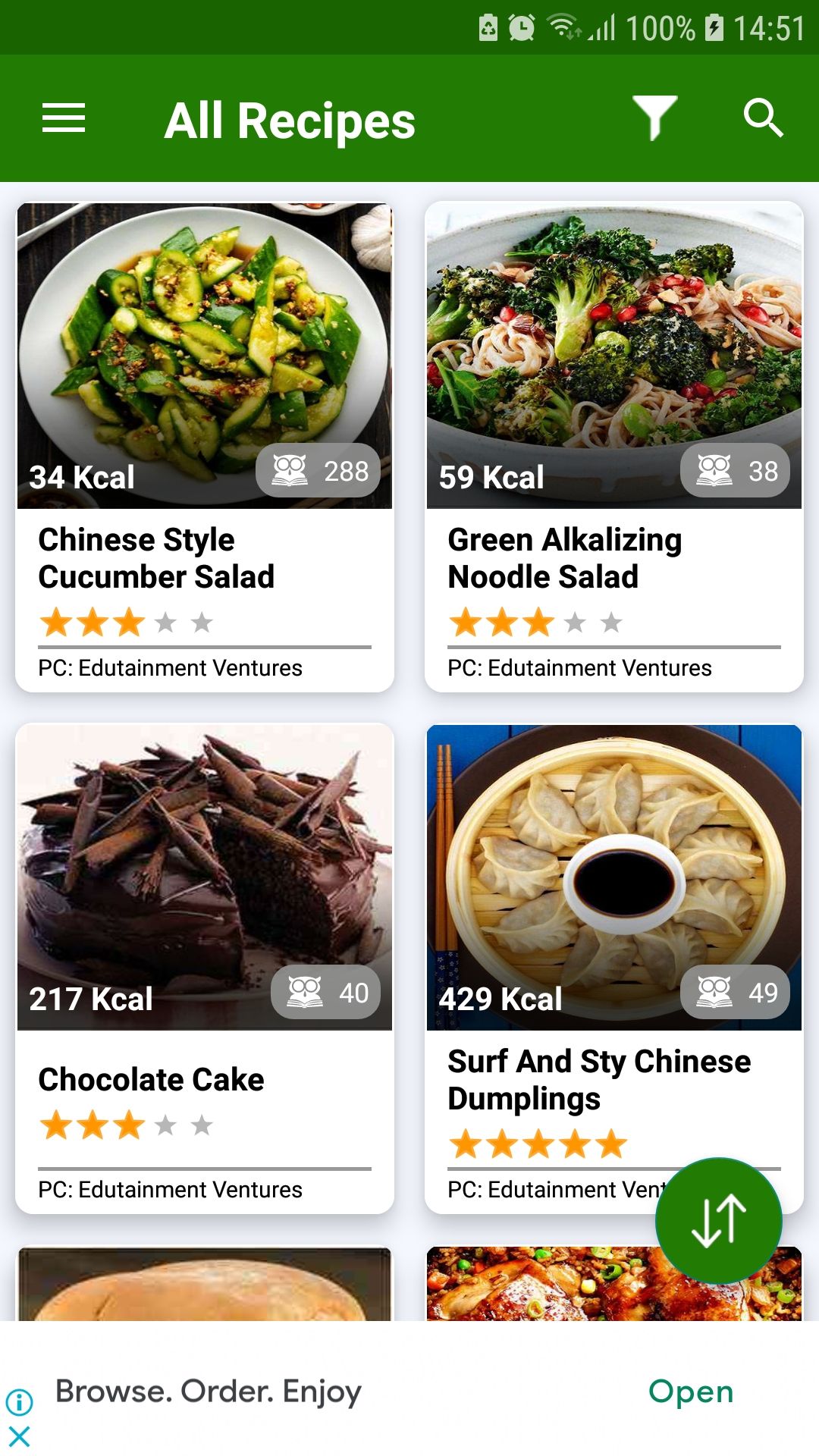A user's cell phone screen displays a webpage from AllRecipes.com. The phone shows 100% battery life, the time as 14:51, an alarm icon, and one bar of network signal. The top of the webpage features a dark green banner with the text "All Recipes" in white. To the right of the banner are filter and search icons, while to the left is a menu icon represented by three horizontal bars. 

The webpage displays several recipes, each within a rectangular box that includes an image, calorie count, and the recipe title. At the top left, there is an image of a "Chinese-Style Cucumber Salad" served on a white round ceramic plate. To the right, the "Green Alkalizing Noodle Salad" is shown with a calorie count of 59 per serving and an accompanying image. Both these recipes have three out of five stars.

Below, there’s an image of a "Chocolate Cake," with a slice visibly taken out, carrying a caloric value of 217 per serving and a three-star rating. To the lower right, "Surf and Style Chinese Dumplings" are displayed with a five-star rating and 429 calories per serving. Two more recipes are listed underneath, but they are partially cut off at the top.

At the bottom of the screen, a banner reads "Browse, Order, Enjoy," alongside a blue "Open" button. Up and down navigation arrows are displayed within white circles outlined in green.